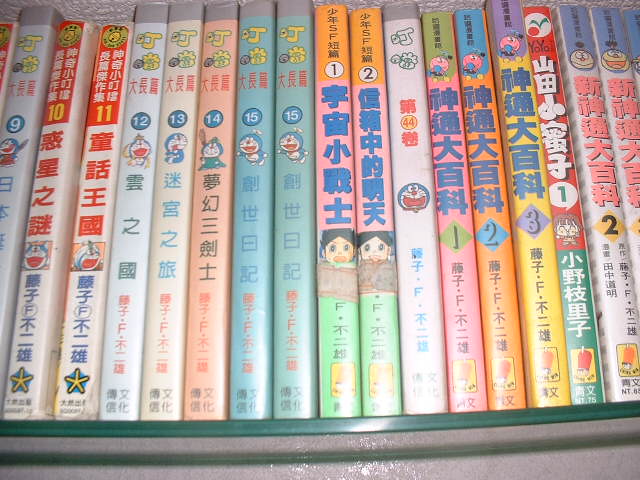The image showcases a landscape-oriented photograph of a row of 17 books with their spines facing outward. Each book features Asian writing, likely Japanese or Chinese, and is meticulously arranged on a thin glass shelf outlined in green, set against a gray wall. The books are vibrantly colored, with spines in various hues of white, salmon pink, light blue, red, orange, and yellow. They display numbers in typical Western numerals: starting from 9 and sequentially going up to 16, then cycling back to 1 and 2, followed by a number 44, another sequence from 1 to 3, and ending with a cut-off book appearing to be numbered 3. Some of the spines feature anime illustrations. The detailed and colorful arrangement provides a vivid and organized display of the collection.